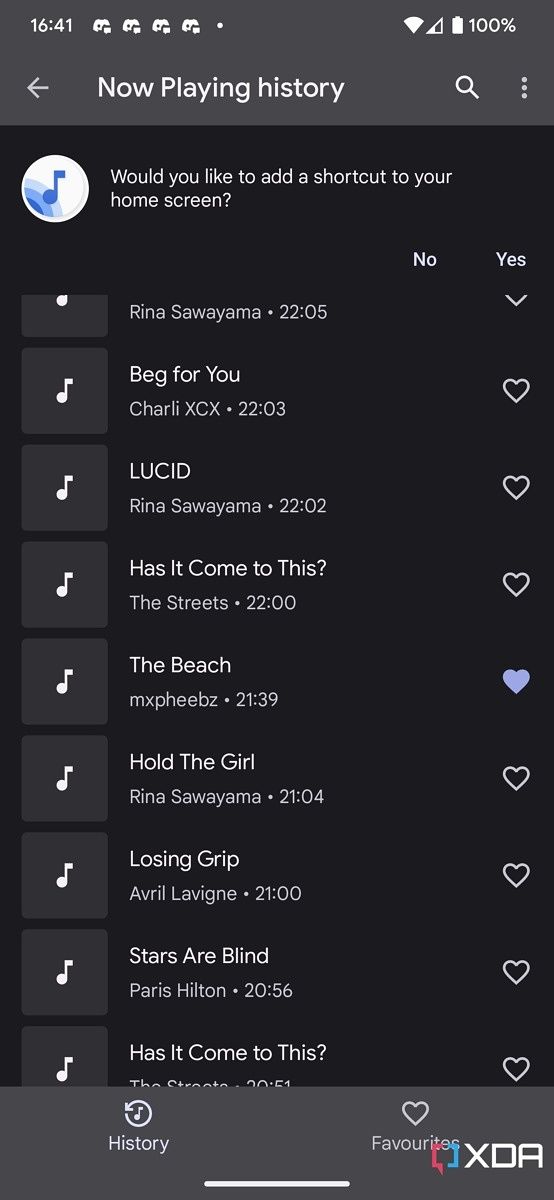The image is a screenshot taken from a cell phone, featuring a music player interface against a solid black background. At the top of the screen, a title bar displays "Now Playing History" with a left-pointing arrow on the far left and a magnifying glass icon on the far right. The upper left corner shows the current time, "41," along with an icon of a video game controller. The upper right corner indicates that Wi-Fi is enabled and the battery is fully charged at 100%.

Below this, there's a white circle with a blue musical note icon. Next to it, a message reads, "Would you like to add a shortcut to your home screen?" with two options: "No" and "Yes."

The music playlist displayed below includes several tracks:
1. "Raina Sawayama" with a duration of 22 minutes and 5 seconds.
2. "Beg For You" by Charli XCX, 22 minutes and 3 seconds.
3. "Lucid" by Raina Sawayama.
4. "Has It Come to This?" by The Streets, 22 minutes.
5. "The Beach" by MXPhebes, 21 minutes and 39 seconds.

To the right of the playlist, there is a blue heart icon.